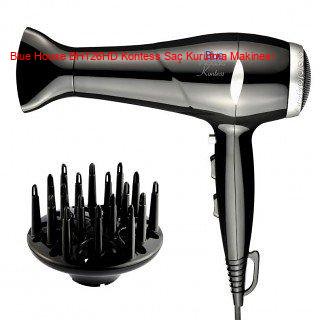The image depicts a detailed view of a hairdryer against a pure white background, giving it a minimalistic yet focused presentation. The hairdryer itself is predominantly black with a few silver components, and it has a compact and somewhat elongated design. The hairdryer's handle features three buttons and a small loop at the bottom for hanging. Additionally, there is a small white section near the top of the handle. Notably, the back end of the hairdryer, where the air intake is located, is silver with a black screen cover.

A distinctive feature of this hairdryer is the presence of red text along its body, which includes brand information and possibly model details, though the exact wording and language are not entirely clear. The text references "Blue House DHT 26 HD KONT SS SAC MAKINE A."

The main barrel of the hairdryer, which expels the air, is pointed to the left, creating a 90-degree angle. This part of the device might be black and silver as well and appears to taper off into a design resembling a crimped Y-shape, likely to direct air in a more controlled manner.

Sitting next to the hairdryer is a detachable diffuser attachment. This attachment is circular with black plastic spikes extending vertically, designed to help distribute air evenly and add lift and body to curls.

The overall impression is of a well-designed, functional hairdryer with a sleek appearance and useful attachments, emphasizing both aesthetic appeal and practicality.